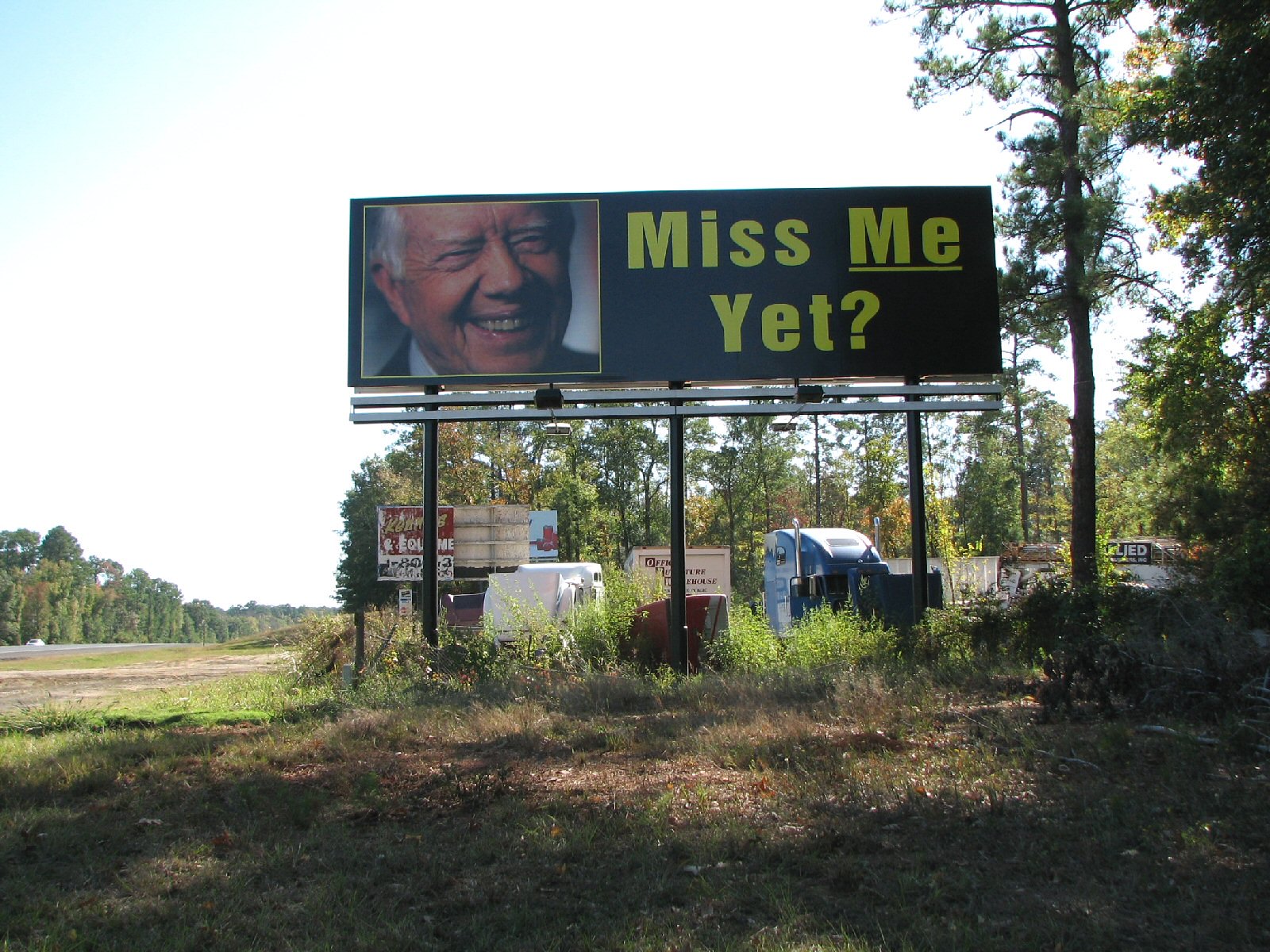The image captures a large billboard set against a fairly sunny, predominantly clear blue sky with some white clouds. The billboard, which has three supporting pillars, features a striking design with a black background and bold yellow block text that reads "Miss me yet?" The word "me" is emphasized with an underline. To the left of the text, there is a color headshot of a smiling, elderly Jimmy Carter, recognizable by his gray hair and Caucasian features. Surrounding the billboard, tall coniferous trees cast their shadows onto the sign, enhancing the scenic outdoor setting.

In the background and to the right of the billboard, there are more tall trees adding depth to the landscape. Below the billboard, a partially visible blue truck with its hood and passenger door open is seen, along with some patches of long grass. A secondary old, weathered billboard with remnants of a torn sign stands behind it. Further details include a white car on the road and what appears to be another truck or camper with an open trunk or hood, emphasizing a rural, roadside atmosphere. This scene gives the impression of a snapshot taken during a voyage through a wooded area alongside a less-traveled road.